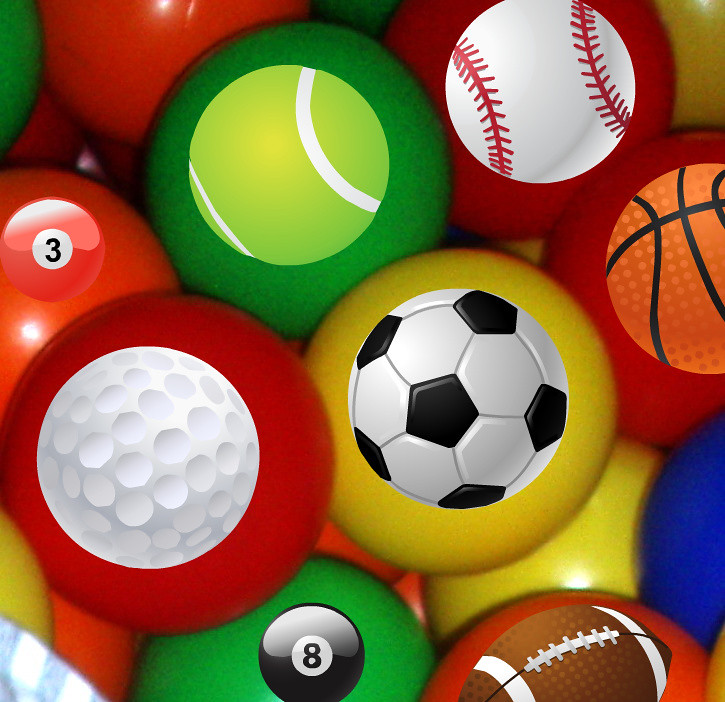The image is a vibrant digital artwork showcasing an array of multicolored plastic balls, reminiscent of those found in a ball pit, overlaid with detailed icons of various sports balls. The photo features red, green, yellow, and blue plastic balls, each adorned with digitally superimposed sports ball icons. Prominently, there is an orange pool ball with the number three, a red ball featuring a golf ball with dimples, a green ball with a yellowish-green tennis ball, and a black eight ball on a green backdrop. Other icons include a baseball with red seams on a red ball, a white and black soccer ball on yellow, a brown American football, an orange basketball, and a traditional black-and-white soccer ball. The art is characterized by its colorful diversity and meticulous overlay of sports ball images on plastic ones, creating a playful and visually engaging composition.